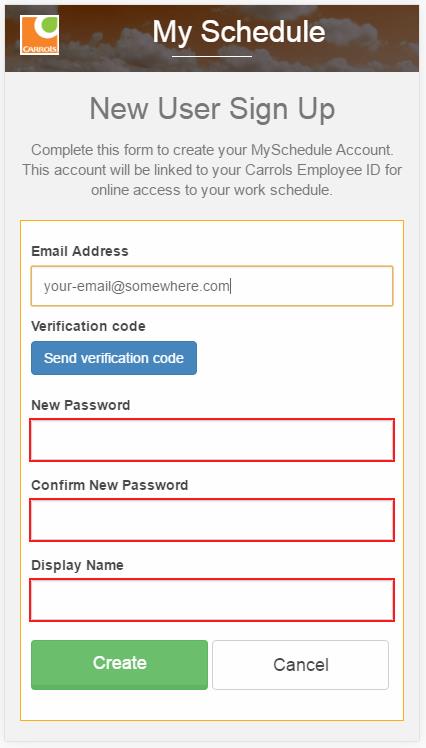The screenshot depicts a web page with a prominent orange background featuring semi-transparent clouds. In the top left corner of the page, there is a square with a white border that has an orange segment in its lower left corner. Inside this square, a white circle encases a smaller green circle. The text "KARROTS" (sic) is displayed in the lower left-hand corner of the square.

At the center of the image, bold white text reads "My Schedule" underlined by a white line. Surrounding this, in a dark gray area, are the phrases "New User Sign Up" in dark gray text and "Complete this form to create your my schedule account. This account will be linked to your Carols employee ID for online access to your work schedule." in regular gray text, suggesting a correction in the spelling from 'KARROTS' to 'CAROLS'.

Below this introductory text, there is a yellow-bordered sign-up form. The form fields are detailed as follows:

- **Email Address**: This label is in bold black text, with a rectangular input field outlined in gold that has the placeholder text "your-email@somewhere.com" in gray.
- **Verification Code**: Bold black text above a button that is dark blue with bold white text reading "Send Verification Code".
- **New Password**: Labeled in bold black text, followed by a rectangle with a red border for the input field.
- **Confirm New Password**: Similarly, labeled in bold black text with a red-bordered rectangle for the input.
- **Display Name**: Also in bold black text with a red-bordered rectangle for the input.

Finally, two buttons are available at the bottom of the form: a green button with white text that says "Create" and a white button with black text that says "Cancel".